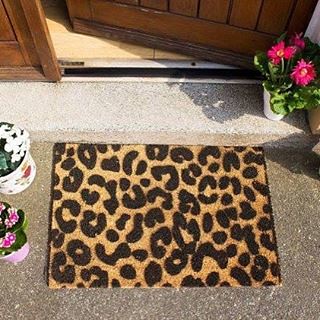This image captures a rectangular doormat with a cheetah or leopard print design, characterized by a beige background adorned with black markings, placed on a grey surface resembling a street sprinkled with little white specks. The scene is set in front of a slightly open dark brown wooden door, showcasing the wood grain and planks, with a silver and black weather stopper visible at the bottom. Inside the door, the yellow tile flooring of the home is discernible. Surrounding the doormat are three plant pots of varying sizes, vividly colorful with pink, red, white, and hot pink flowers. On the right side, a larger pot boasts bright pink flowers with green stems and leaves. To the left, two smaller pots display light pink flowers tinged with purplish hues and another with white flowers, one pot adorned with a small drawing. The sunlight casts shadows onto the front door and the interior, enhancing the overall warm and inviting atmosphere.